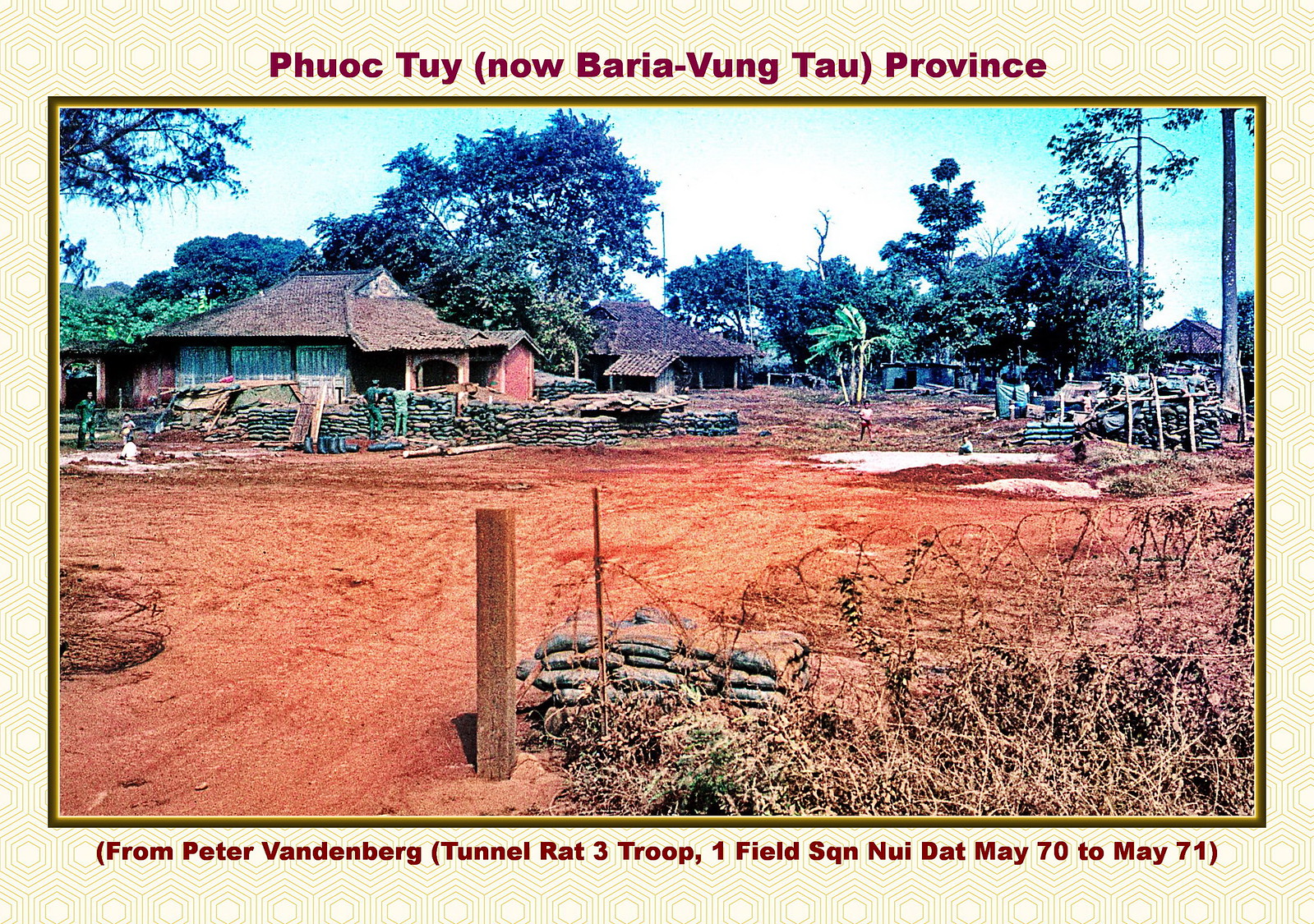This photograph, likely taken between May 1970 and May 1971 in what is now Ba Ria-Vung Tau Province, Vietnam, depicts a rural wartime landscape. It is bordered by a tan, textured frame and features red text at the top that reads "Phuoc Toi, now Ba Ria-Vung Tau Province." At the bottom, it is captioned "From Peter Vandenberg, Tunnel Rat 3 Troop, 1 Field SQN, Duy Dat, May 70 to May 71." 

The central focus of the image is a large, red dirt field flanked by three small structures—presumably houses or huts with thatched roofs—on the left side. These structures are set against a backdrop of lush green trees under a clear blue sky, suggesting the photograph was taken outdoors in the middle of the day. In the foreground, numerous stacks of sandbags are visible, likely serving as fortifications, hinting at the military presence and activity in the area. Additionally, there are people in military uniforms walking around in the background, adding a sense of everyday life amidst the wartime setting. The scene captures a moment in Vietnam's history, offering a detailed glimpse into its landscape and the people during this period.